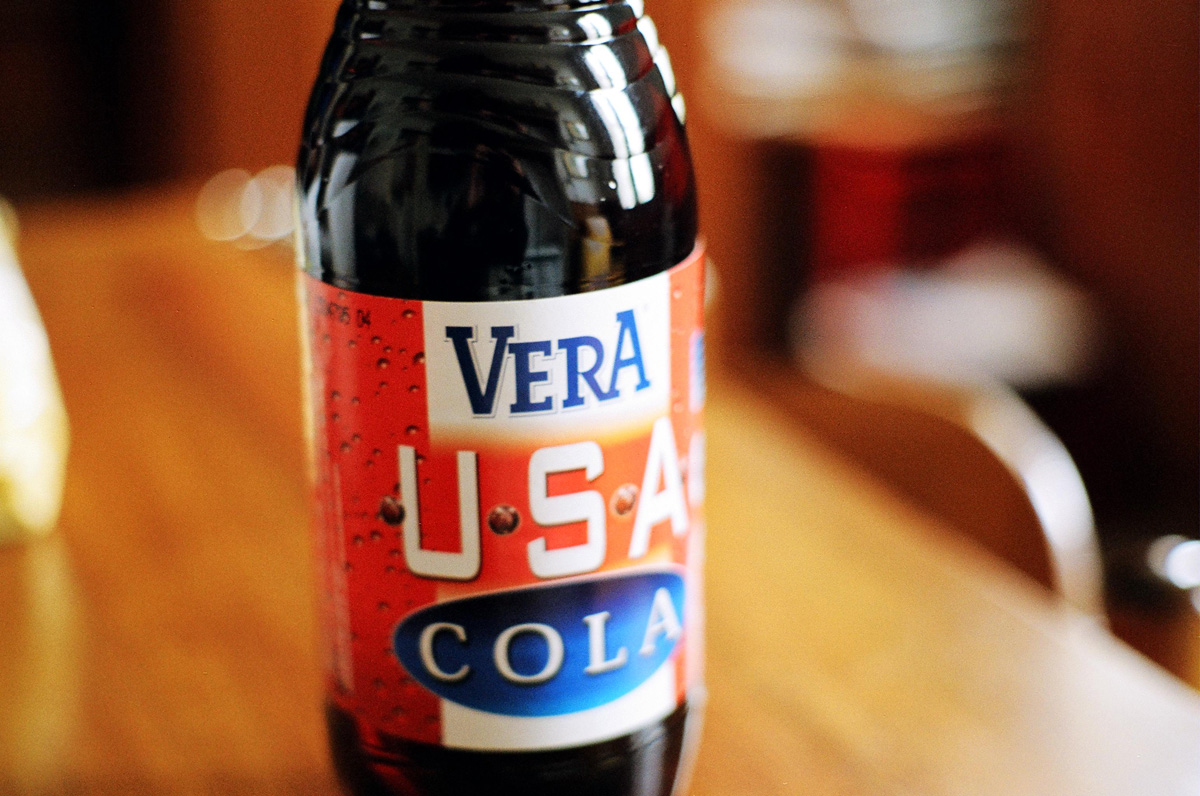This detailed close-up photograph showcases a bottle of "Vera USA Cola." The image is in landscape orientation and captures the bottle prominently. The label features "Vera" in blue fonts, "USA" in white fonts against a red background, and "Cola" in white fonts against a blue background. The liquid inside the bottle is a rich, dark, nearly black color. The bottle is placed on a light brown wooden table, adding a warm contrast to the dark soda. The background is artistically blurred, highlighting the bottle's sharp details, while a few indistinct white and red shapes subtly populate the out-of-focus area.